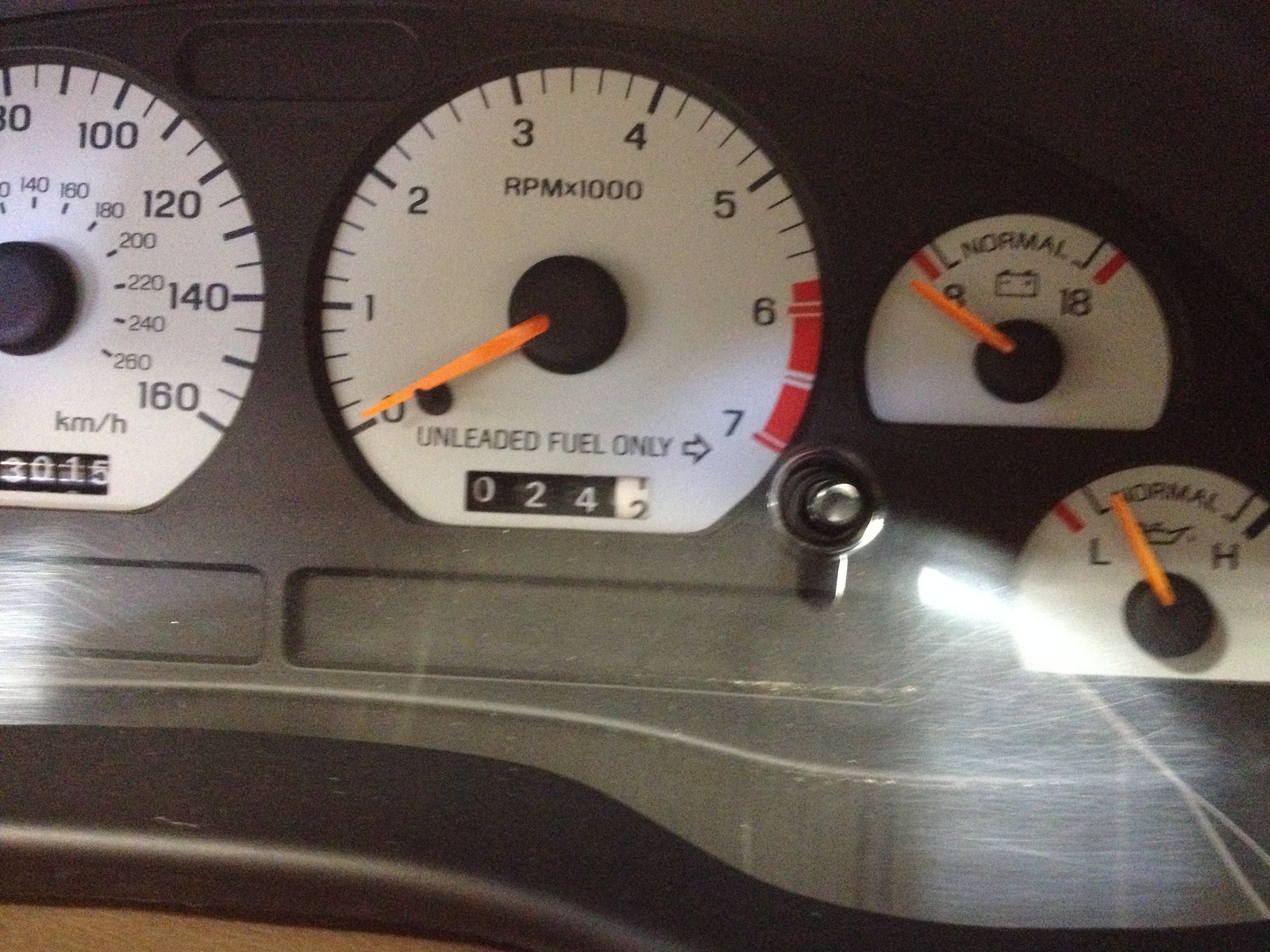The photograph captures the dashboard of a vehicle featuring several important gauges. On the left side is a partially visible speedometer marked in increments up to 160 miles per hour. Centered prominently on the dashboard is the RPM gauge with a label reading "RPM x 1000" and "unleaded fuel only," and it shows a reading of 0 RPM. The trip meter below this gauge displays a mileage of 0242. To the bottom right, there are two smaller gauges: the first one indicates the battery level, marked from 0 to 8, with the needle pointing at 0, suggesting the vehicle might be off. The second gauge monitors the oil level, marked from 'L' (Low) to 'H' (High), with the needle leaning towards 'L'. The gauges feature an orange needle, and the dashboard itself is a gray background. Overall, the image provides a clear and detailed view of the vehicle's essential monitoring instruments.